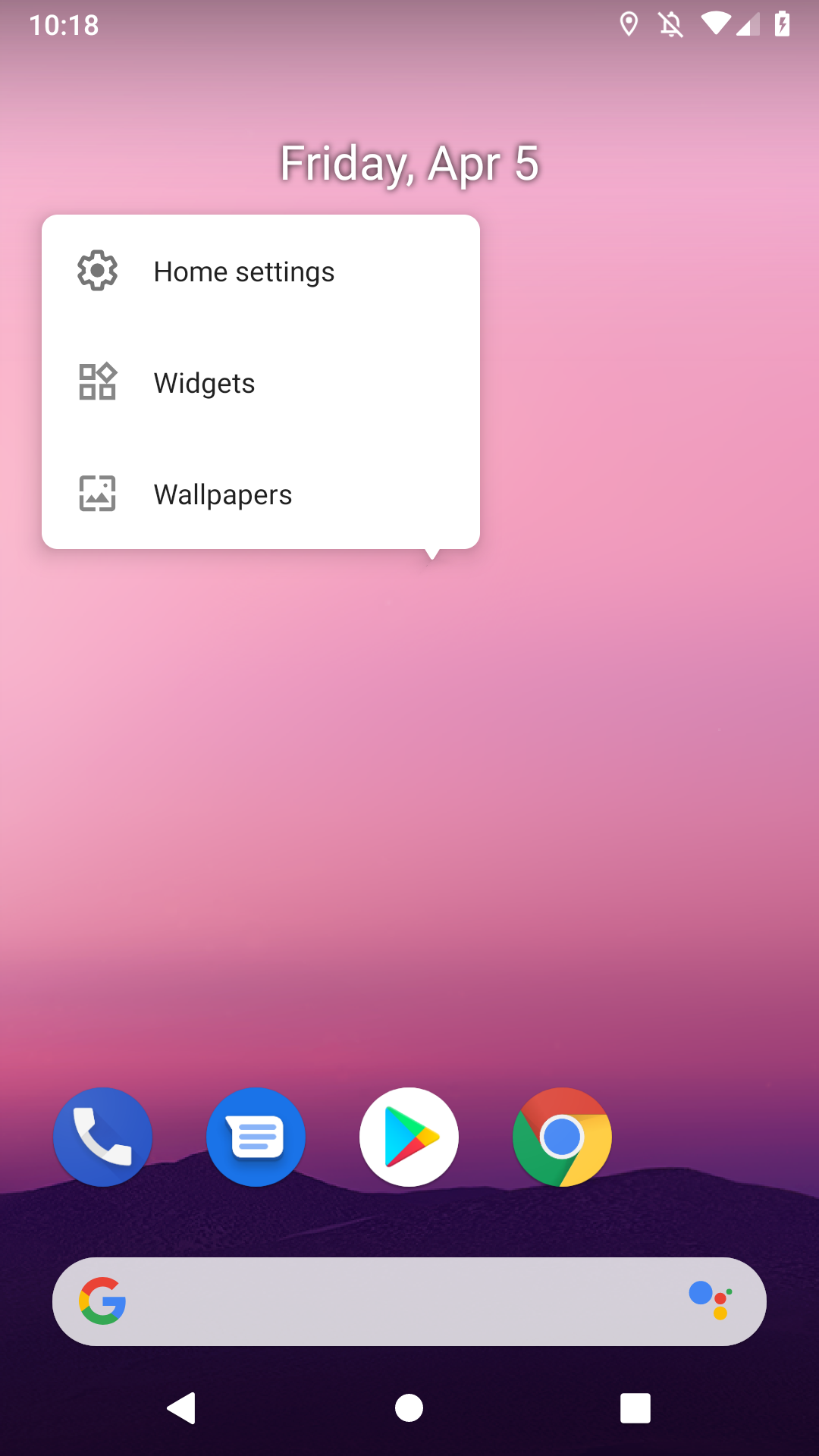A detailed screenshot of an Android phone's home screen, featuring a purple background with a dark purple silhouette of mountain tops at the bottom. In the top left corner, the time is displayed in white, and the top right corner shows icons for location enabled, sound turned off, active Wi-Fi connection, phone signal strength, and battery status. Below the icons, centered on the screen, the date is displayed in white, reading "Friday, April 5th." A pop-up menu appears slightly left of the center, featuring a small white box with options for "Home settings," "Widgets," and "Wallpapers." Towards the bottom of the screen, there are four prominent circular icons: a large round blue icon with a telephone symbol representing the phone app, a lighter blue circle with a chat bubble symbol for text messages, the Google Play icon inside a white circle, and the Google Chrome logo. Below these icons, a search bar is situated with the Google "G" logo on the left and multicolored bubbles symbolizing the voice search or send function on the right.